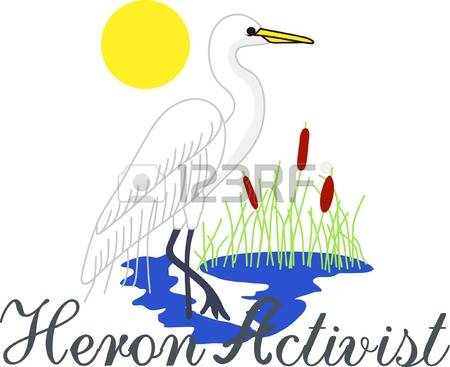The computer-generated graphic art centers on a white heron with long black legs and a striking yellow beak, standing gracefully on one leg in stylized blue water. Surrounding the bird are thin green lines representing grass and cattails, characterized by their distinctive brown fuzzy tops. A bright yellow circle, symbolizing the sun, is positioned behind and to the left of the heron, adding contrast to the predominantly white background. The scene is marked by a "Heron Activist" inscription in elegant black cursive script across the bottom of the image. A conspicuous 123RF watermark with a gray camera icon and copyright symbol is placed in the center, reminding viewers of the image's source. This vibrant and detailed illustration, possibly intended for a bumper sticker, embodies environmentalist themes and a love for nature.